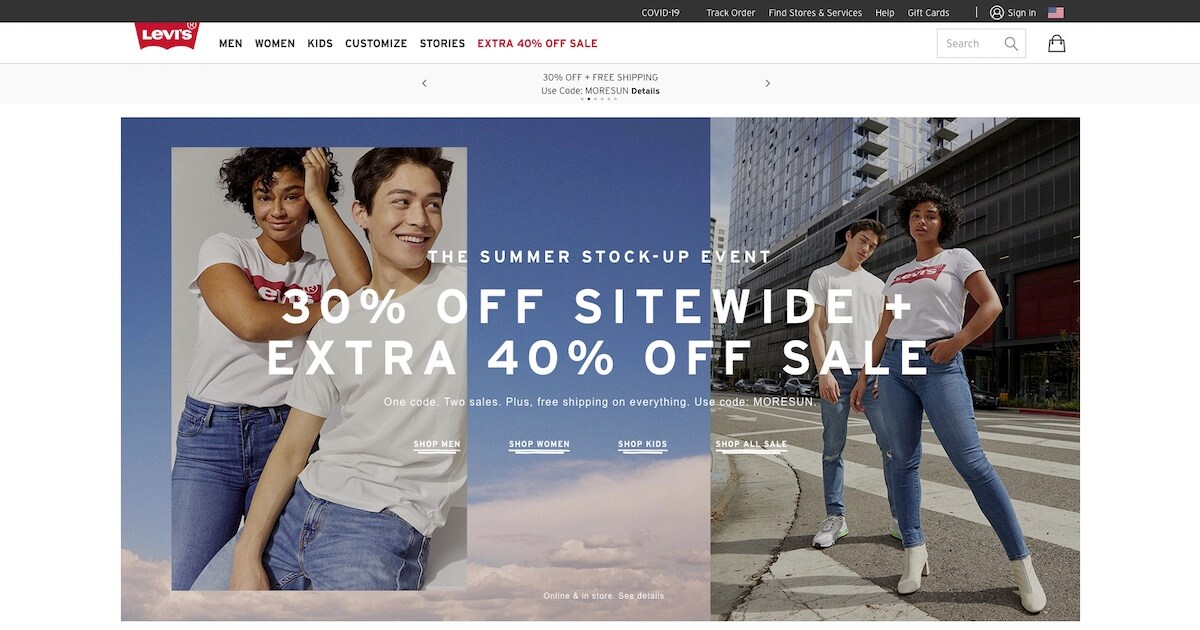Screenshot of the Levi's Online Store: 

At the top of the page, a sleek black banner spans across, featuring essential navigation options such as COVID-19 updates, track order, find stores and services, help, gift cards, and sign in, accompanied by an American flag icon. Directly underneath, the iconic Levi's logo is prominently displayed, followed by a menu bar with categories for Men, Women, Kids, Customized, Stories, and a special "Extra 40% Off Sale."

Highlighted just below the menu, there's a bold promotional message offering 30% off plus free shipping with the code "MORE SUN." Dominating the center of the screen is a wide, eye-catching rectangular photograph showcasing a young woman and young man in a stylish, casual setting. The image is split into two side-by-side photos.

On the left side, a young woman with short dark hair and dark skin stands poised. She strikes a unique pose with her right arm bent at the elbow and curving in front of her while her left arm is bent, with her hand resting on top of her head. She wears a white t-shirt emblazoned with the Levi's logo, paired with blue jeans. To her right, seated, is a young man with short dark hair, appearing to be of Asian descent. He gazes off to the right with a cheerful smile, dressed in a plain white t-shirt and blue jeans, complementing the woman's effortless style.